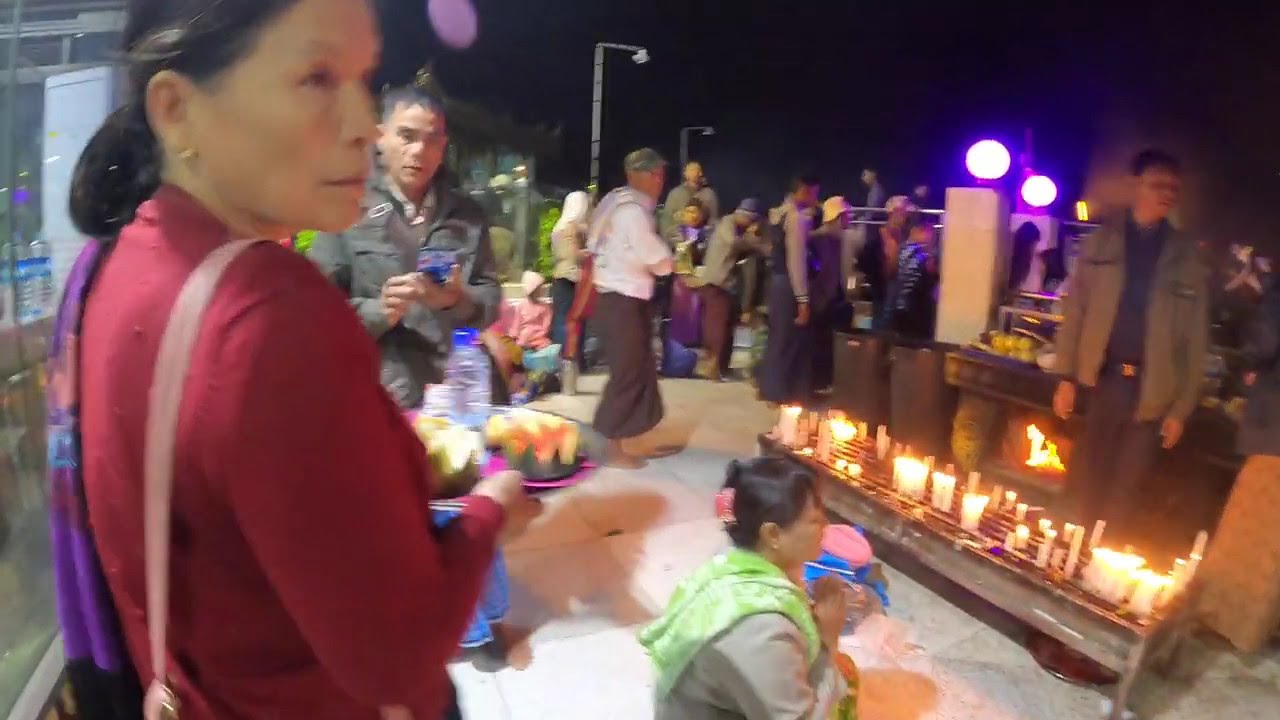The image depicts an outdoor nighttime gathering, possibly in an Asian nation, distinguished by a dark black sky. To the left, a woman in a red long-sleeve shirt stands out, adorned with studded earrings, a purple scarf draped over her left shoulder, and a pink purse on her right shoulder. She cradles a silver tray laden with pink plates filled with cut melons alongside a water bottle with a blue cap. In front of her is an altar-like setup covered with lit pillared candles, illuminating the scene. There's a man behind the candles, clad in an olive-colored jacket and navy blue attire. To the right, a woman dressed in green is crouched down, adding to the atmosphere of this celebratory gathering, as more people gather in the background, casting an ambiance of communal warmth and festivity.